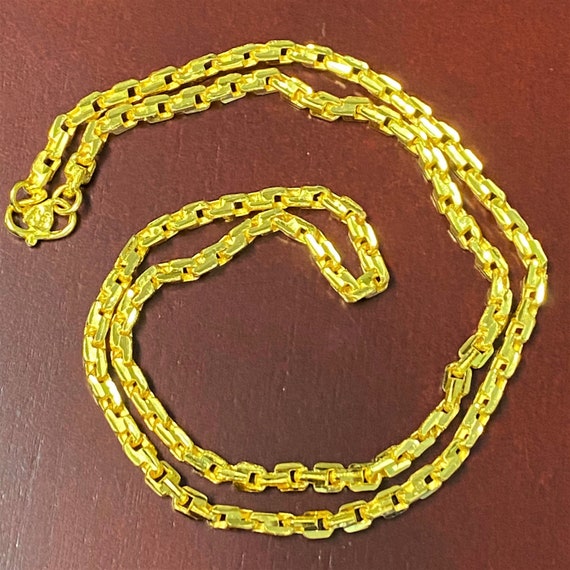This photograph features an intricately detailed and substantial gold chain necklace, lying on a textured brown background that appears to be wood or painted wood. The necklace, made of large interlocking rectangular links with openings in the center, has a prominent oval clasp at one end, which secures the two ends of the chain together. The chain is arranged in a neat, circular pattern, reminiscent of a maze or a coiled snake, curling inward to form a shape similar to a backward number six. The links are three-dimensional and notably do not lie flat, giving the chain a clunky yet beautifully displayed appearance. The necklace, which looks shiny and bright, is approximately 16 to 18 inches in length and positioned on a burgundy-tinted surface, enhancing its lustrous gold hue.